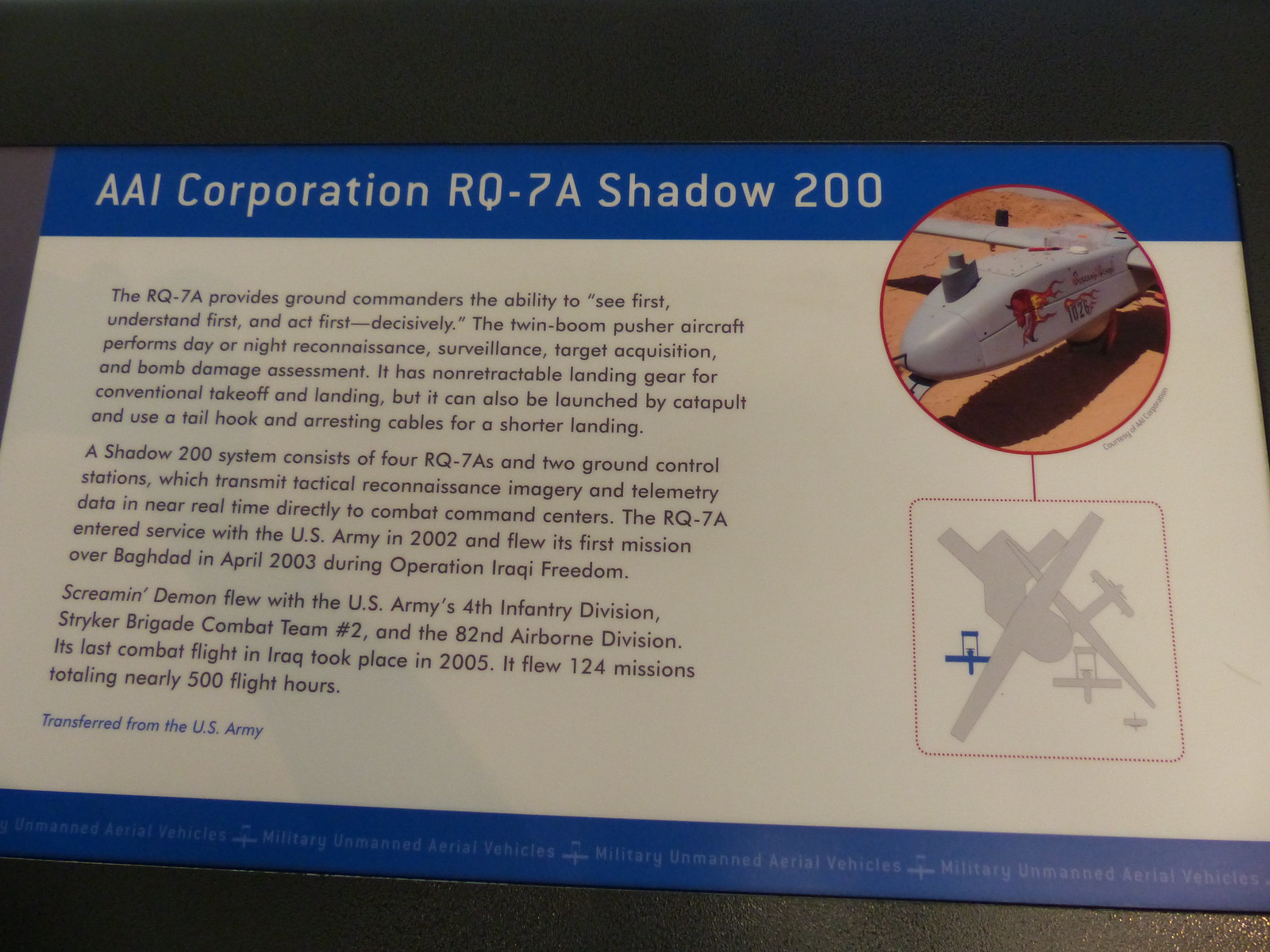The image showcases an informational plaque or display panel about the AAI Corporation RQ-7A Shadow 200, likely situated in a museum or exhibit. Dominating the top section of the plaque, a blue bar prominently displays the name "AAI Corporation RQ-7A Shadow 200." The right side features a close-up circular image of the nose section of this military drone, highlighting its white exterior. Beneath this, a square gray-shaded diagram presents detailed aspects of the drone's design. Centrally placed, small black print, organized into three paragraphs, offers comprehensive information about the RQ-7A's capabilities and service history. The text elaborates on the drone's role in providing ground commanders with critical reconnaissance, surveillance, target acquisition, and bomb damage assessment capabilities, both day and night. It details the aircraft’s innovative non-detectable landing gear for conventional landings as well as its ability to use a catapult launch and tail hook for shorter landings. The description outlines the Shadow 200 system, consisting of four RQ-7A drones and two ground control stations that transmit real-time tactical reconnaissance imagery and telemetry data directly to combat commanders. The panel notes the drone's entry into service with the U.S. Army in 2002 and its first mission over Baghdad in April 2003 during Operation Iraqi Freedom. At the very bottom, the plaque indicates that the display was transferred from the U.S. Army. The entire display is presented against a white background.